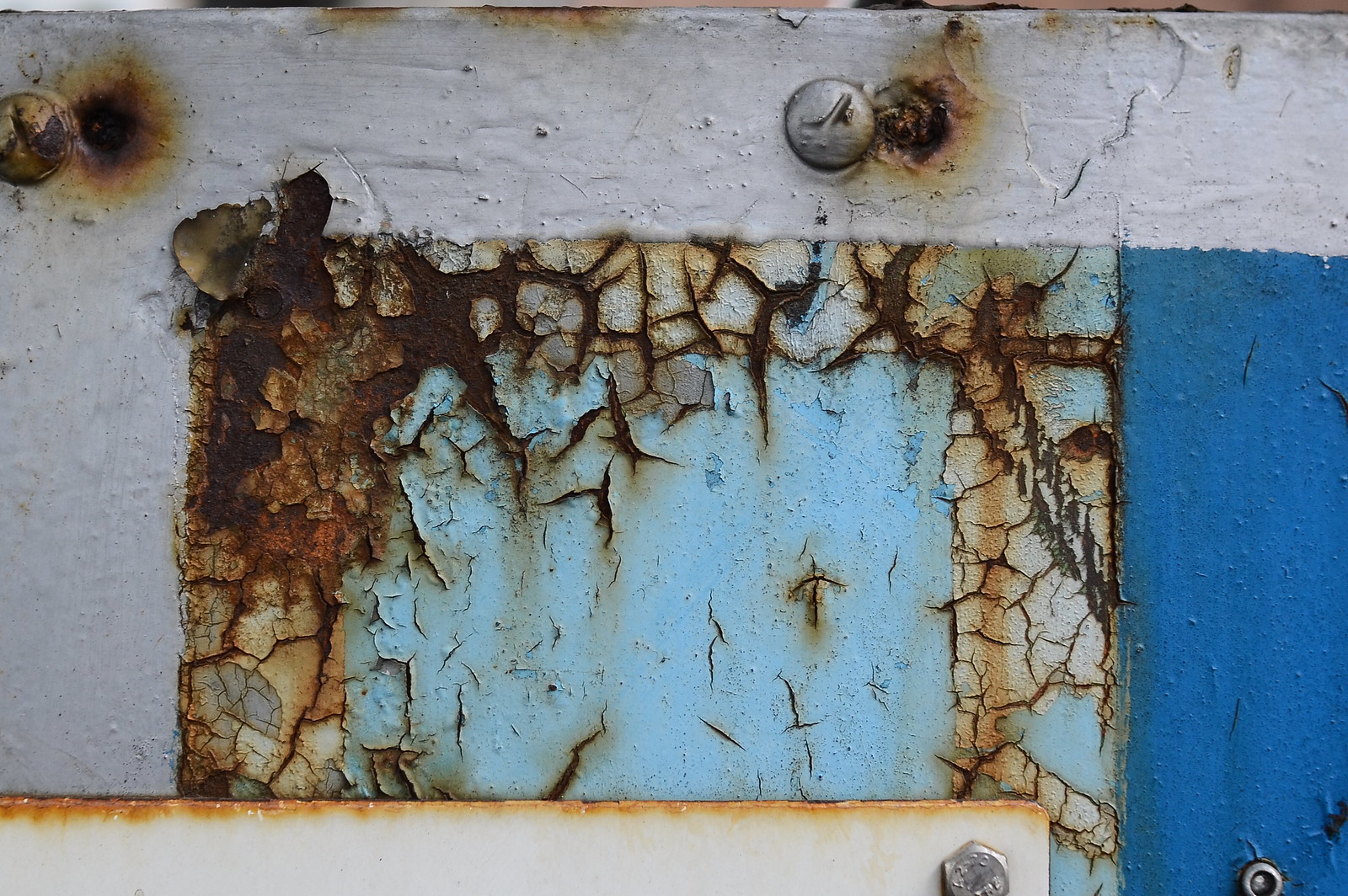The image captures a close-up of a very old and weathered metal structure, heavily damaged by rust and time spent exposed to the elements. The paint, in fading and chipped layers of white, light blue, and dark blue, is peeling away to reveal extensive rust underneath. Different types of bolts secure multiple metal plates, including Allen bolts, round bolts, and hex nut bolts. The top left features a rusty design with notable rust damage around the screws. Similarly, the middle right shows rust damage around another screw. At the bottom, there's a white panel detailed by a metal screw on the right side, while the middle of the image showcases a deteriorating blue panel. Edges of the structure reveal metallic cutouts and additional paint chipping, especially on a blue rectangle with a bolt in the bottom right. A white strip runs horizontally at the top and descends on the left, also marred by rust damage. Cracks and holes in the paint expose the red rusted metal beneath, evidencing the extensive wear and neglect over many years. Overall, the photo vividly displays the corrosive effects of time on this metal object, with every detail underscoring its advanced state of decay.